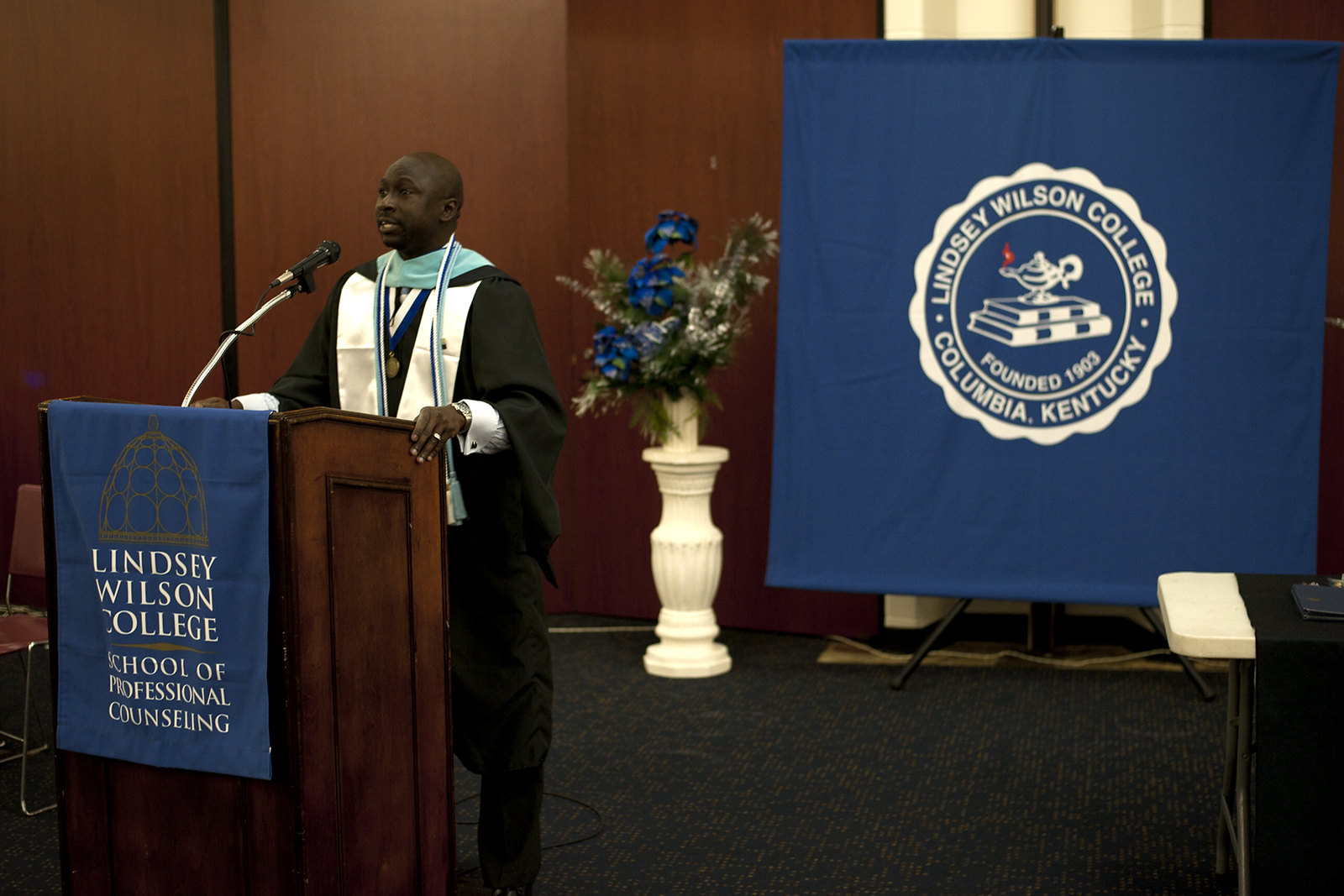In the image, a man with dark skin stands behind a brown wooden podium adorned with a blue banner that reads "Lindsay Wilson College, School of Professional Counseling" in white letters. He is almost bald and is wearing a layered academic robe featuring a black gown with a blue sash and a blue scarf. Positioned in front of him is a microphone, suggesting he is delivering a speech, possibly at a graduation ceremony. The setting appears to be formal, likely at Lindsay Wilson College.

To the right of the podium stands a vase with flowers on a stand, adding a touch of elegance to the scene. Nearby, a poster displaying the text "Lindsay Wilson College, Columbia, Kentucky, founded in 1903" with a logo that includes an image of a bird and books is visible. The background is divided into a deep brown wall on the top half and a dark-colored carpet on the bottom half. The color palette of the image includes shades of blue, white, brown, green, black, light blue, and gold, providing a rich yet somber atmosphere for the occasion.